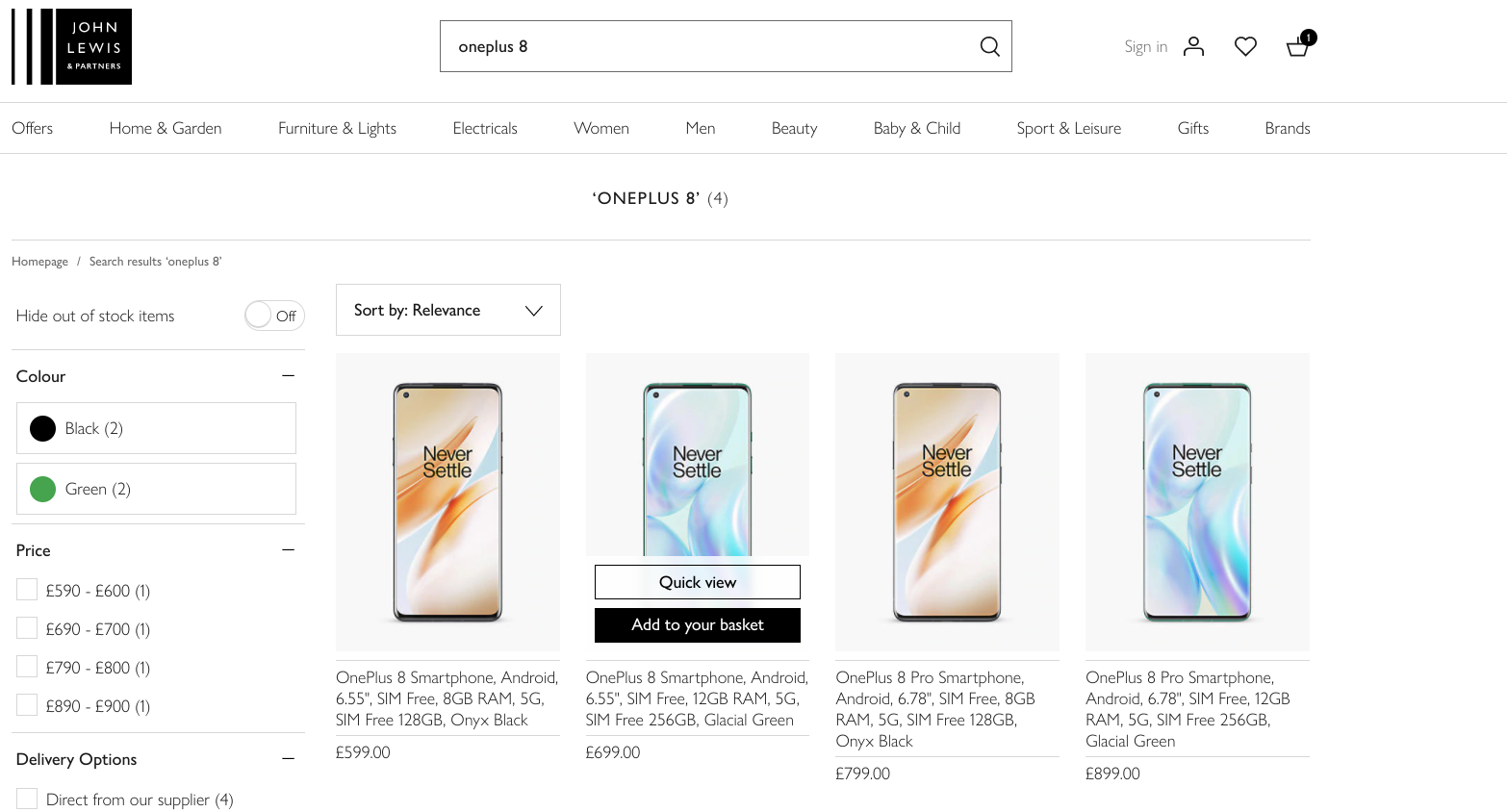This image showcases the John Lewis website. In the upper left-hand corner is the John Lewis logo, designed within a black square with varying line lengths beside it, creating space and edge effects. Below the logo, the text "John Lewis" is displayed with some additional, less legible writing underneath. To the right of the logo, there is a search box containing the phrase "OnePlus 8," typed as "O-N-E-P-L-U-S space 8," accompanied by a magnifying glass icon indicating the search function. Further right, there are options to "Sign In," along with icons for a user profile, a heart (possibly for favorites or wishlists), and a shopping cart with a black circle on its top right corner, likely indicating the number of items in the cart.

Below this primary navigation area, there is a horizontal menu with categories including Offers, Home and Garden, Furniture and Lights, Electricals, Women, Men, Beauty, Baby and Child, Sport and Leisure, and Gifts. This menu is situated within a white banner.

Centrally focused on the page is a display for the OnePlus 8, featuring four different types of phones. To the left, there is a section for selecting the phone color, with options labeled "Black" accompanied by a black circle and "Green" with a green circle. Below the color selection is the price range with four selectable options, and a section for delivery options. A sorting option labeled "Sort by Relevance" is also present.

Each phone is prominently displayed with the brand's tagline "Never Settle." The second phone display slightly differs and includes options for a "Quick View" and buttons for "Add to your Basket," highlighted for easy interaction.